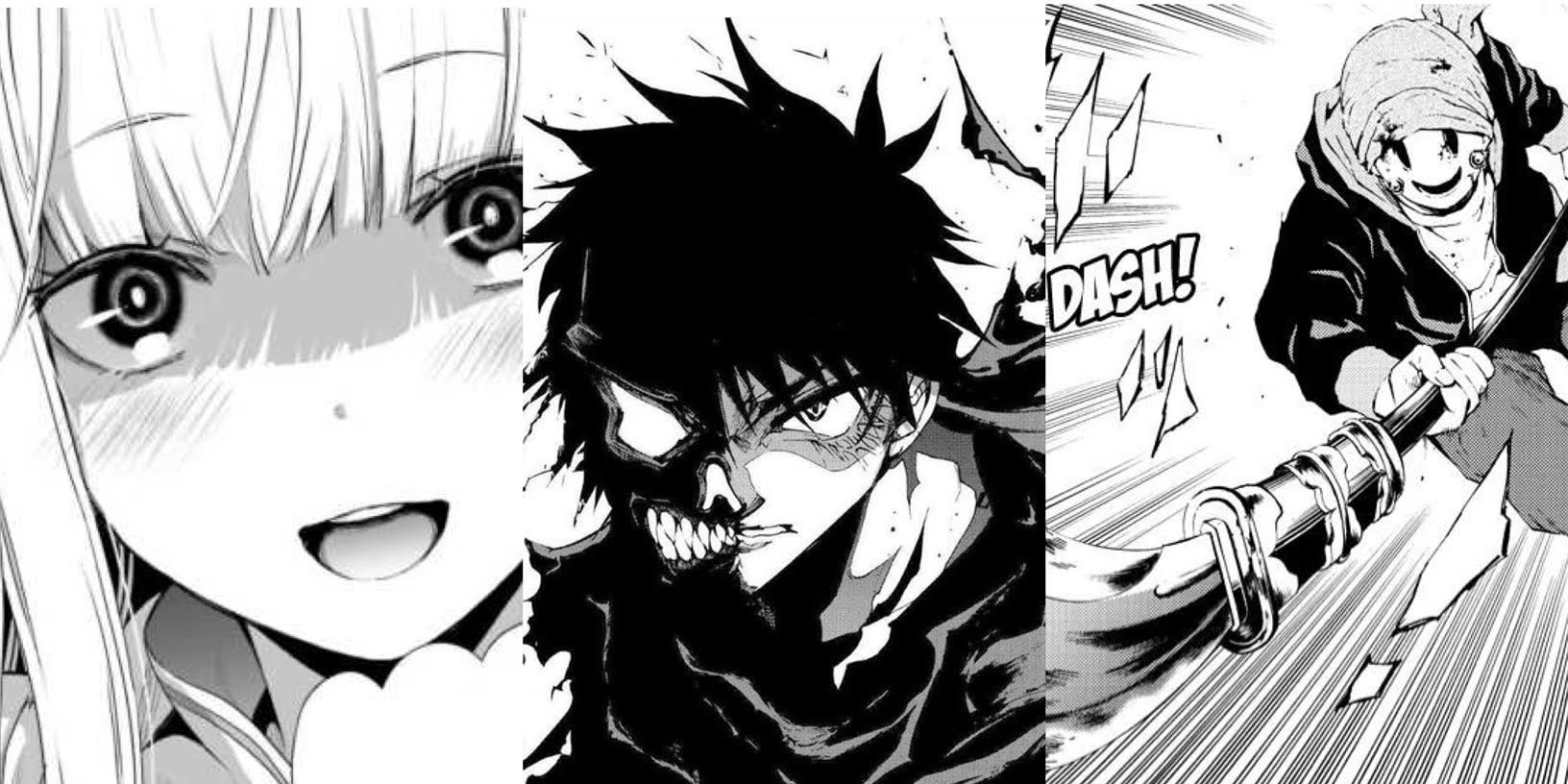The manga-style artwork is divided into three distinct panels, rendered in black and white. The left panel presents a close-up shot of a young woman's face, characterized by her large, expressive eyes and long bangs cascading over her forehead. Her mouth is open, which could suggest a smile or an expression of shock, and subtle shadows add depth to her features. In the middle panel, a man is depicted with a stark contrast between the two halves of his face; one side appears normal with black hair, while the other is grotesquely transformed, resembling a demonic figure with dark, shadowy features, sharp teeth, and a missing eye, evoking comparisons to a Halloween ghoul or the character Two-Face. The right panel shows a dynamic scene where a character, clad in a black jacket and scarf, is charging forward with a broom extended in front of them. The action is emphasized by the word "Dash!" in white text, suggesting a fast and determined movement.